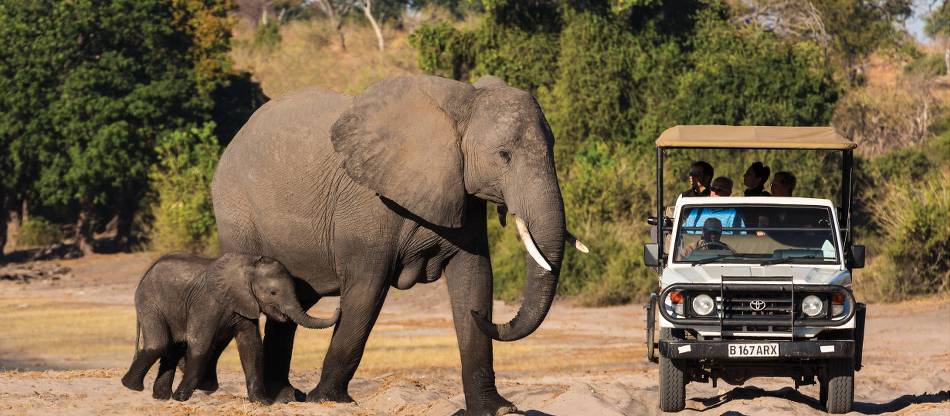This is a detailed photograph of a serene safari scene set in the wild outdoors, showcasing a captivating moment between wildlife and humans. In the foreground, a majestic mother elephant and her baby elephant are walking across a dry, light brown patch of soil from left to right. The tranquil setting is bathed in sunlight, highlighting the elephants as they make their way.

To the right of the frame sits a white jeep, identifiable as an English-style vehicle, with its steering wheel on the right side, and carrying the license plate number B167ARX. The jeep features a yellow fabric canopy, providing shade to four passengers standing and observing the elephants with keen interest. An African man is driving the jeep, witnessing the encounter alongside his passengers.

The landscape orientation of the photograph allows for the inclusion of the wide, natural environment. In the background, there are clusters of light green and dark green trees interspersed with brown vegetation, adding depth to the wild setting. The overall scene encapsulates the essence of an African safari, blending the curiosity of human explorers with the majestic stride of two elephants in their natural habitat.